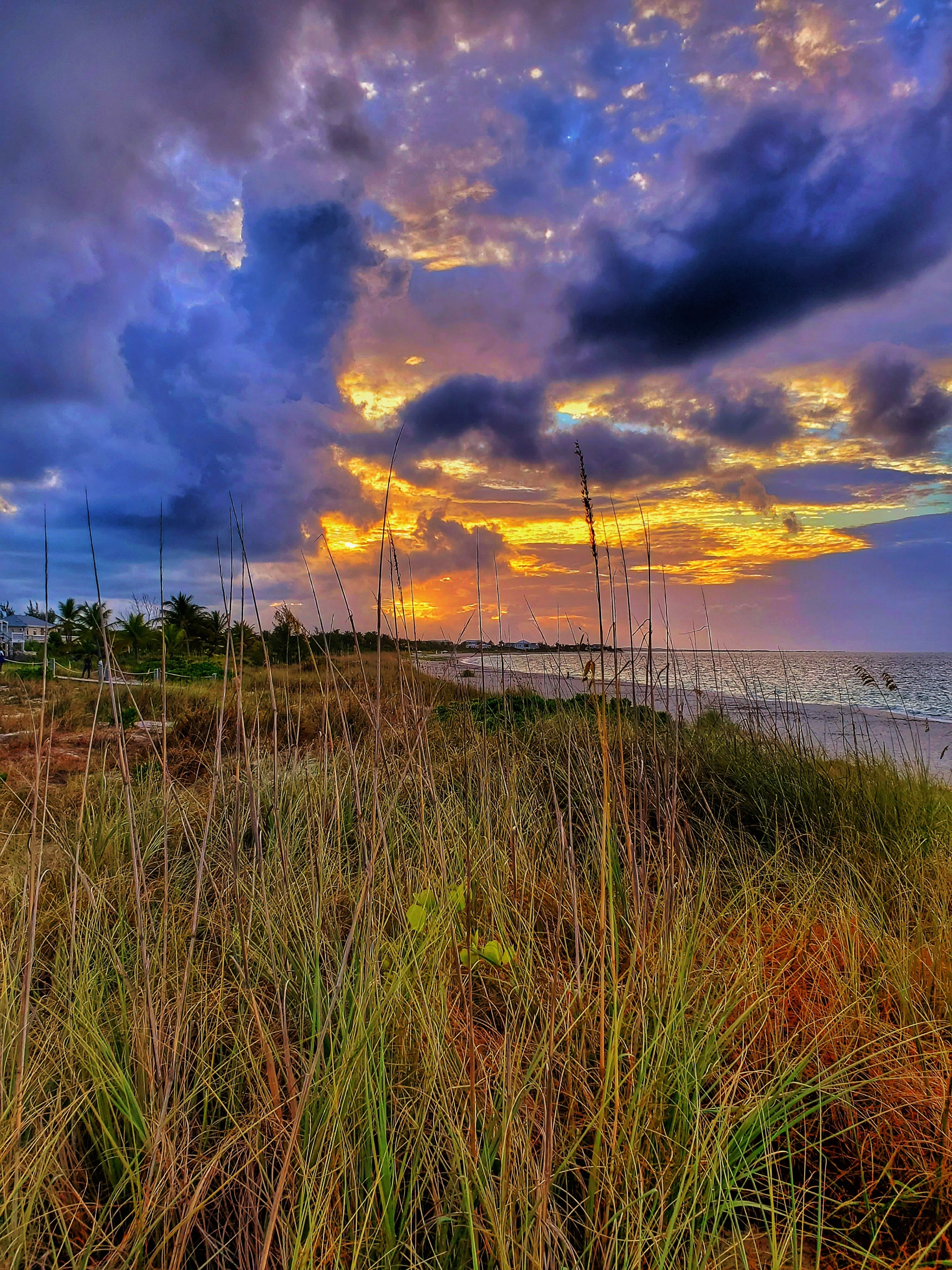This photograph captures a serene beach scene characterized by a lush, grassy foreground with varying hues of green and brown. The tall, swaying blades of grass almost reach the sky, giving a sense of immersion in nature. Beyond the grassy area lies a sandy beach, scattered with wisps of white foam from the water. The water itself remains indiscernible in color but suggests movement and tranquility. In the distance, deep green trees form a line stretching halfway across the horizon from the left, giving way to an unobstructed view of the water on the right.

On the far left of the horizon, a small house nestles among the greenery, adding a touch of human presence to the otherwise untouched landscape. Complementing the scene are majestic palm trees, hinting at a tropical or subtropical location. The sky is a spectacular canvas of colors—deep purples, blues, and greys intermingled with vibrant oranges, yellows, and pinks—indicative of either sunrise or sunset. The stunning interplay of colors in the clouds and the sky lends a peaceful and almost magical quality to the scene, enhanced by the absence of any people, ensuring a sense of calm and solitude.